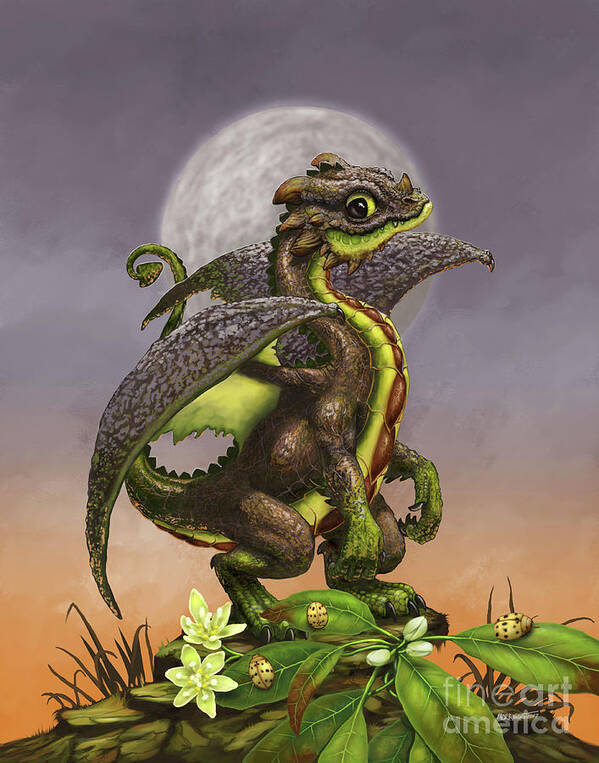This is a detailed digital art piece featuring a baby dragon standing on a stone cliff, set against a striking background. The dragon, which has a rugged rocky texture, is primarily brownish-gray with a green lime-colored underbelly accented by a central brown stripe. It sports large, expansive wings with rough gray exteriors and light green undersides. Its limbs, including its hands and feet, are bright green, and it possesses a curly tail ending in a small, triangular sphere. 

The dragon's gaze is directed toward the viewer, with its head slightly pointed to the right, showcasing a prominent green eye with a large black pupil, complemented by a single horn on its nose and additional horns around the back of its head. Dominating the background, a luminous full moon glows against a purplish-gray and light orange sky, enhancing the mystical ambiance of the scene.

In the foreground, lush green leaves with two white flowers and several off-white, spotted beetles add natural detail. The artwork is subtly marked with transparent white text that reads "Fine Art America" in the bottom right corner, signifying its artistic origin.